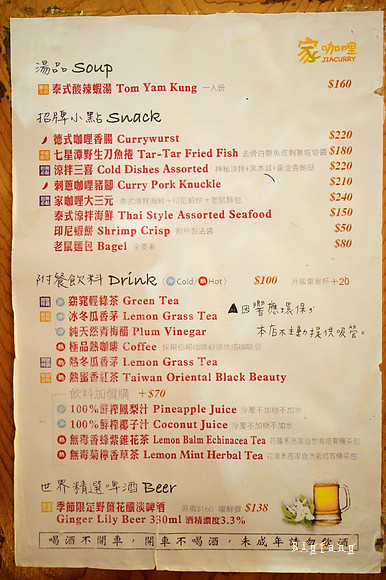The photograph showcases a worn restaurant menu laid atop a light, textured wooden surface. The wood features pronounced grain lines that add visual interest. The menu, an aged and slightly damaged white sheet of paper, shows bent and torn edges, suggesting frequent use.

The menu's headings, such as "Soup," "Snack," "Drink," and "Beer," are printed in black, each accompanied by Chinese characters above the English translations. Beneath these headings, the dishes are listed in red, also starting with Chinese characters followed by English explanations. Various symbols appear next to some dishes, likely indicating attributes such as spice level or temperature preferences.

In the upper right corner of the menu, there is a small, distinct symbol that stands out from the text. The bottom of the photograph features a white watermark stamp, with non-English characters, adding a layer of authenticity and cultural context to the image.